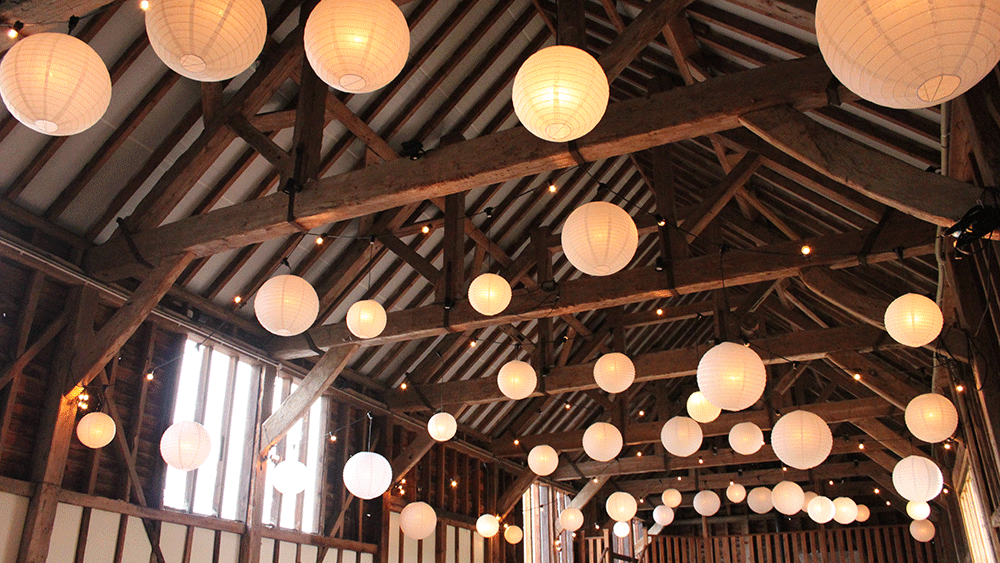This horizontal rectangular image captures the interior of what appears to be an event hall or a rustic barn, possibly used for weddings or parties. The roof features exposed large mahogany wood rafters that extend across a vaulted ceiling, forming a pointed peak at the center. The roof itself is likely metallic, resembling tin, and there is no internal ceiling, allowing a clear view of the intricate framing. The walls mirror the roof's structure, with dark brown beams contrasting against the lower sections painted white. Suspended from the rafters are numerous spherical lights, resembling white Chinese lanterns the size of beach balls or basketballs. These lanterns, about 20 to 30 in number, are distributed randomly throughout the space, casting a warm glow and contributing to the venue's picturesque atmosphere. Most lanterns are homogeneous in size, with a few slightly smaller, creating a visually appealing and festive ambiance.